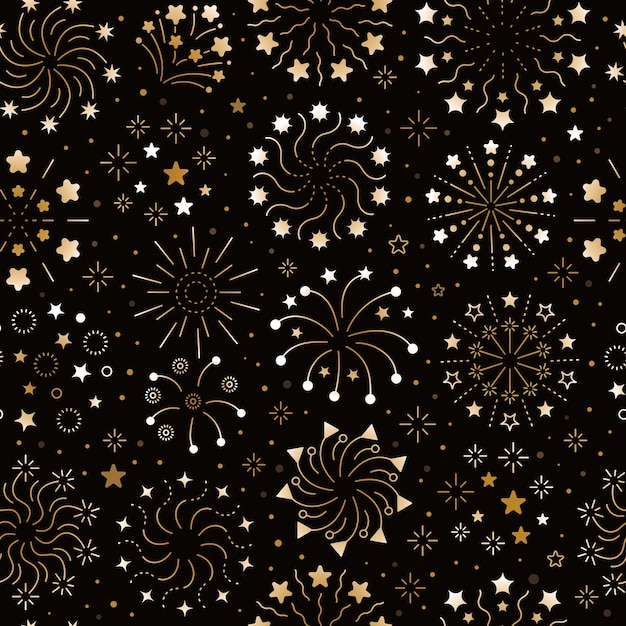This intricate design image on a predominantly black background features an array of swirls and symmetrical patterns, creating a captivating and elaborate display reminiscent of finely illustrated wallpaper or gift wrapping. The composition begins with central black dots, from which lines gracefully swirl and curve. Some lines extend straightforwardly with a star at the end, while others loop and twist akin to the tentacles of an octopus, each adorned with decorative star shapes.

The pattern, appearing meticulously refined by a program like Adobe Illustrator, showcases a dynamic mix of plain shapes in diverse colors, including whites, light browns, golds, and shades of yellow and orange. It achieves a balance between symmetry and subtle asymmetry, ensuring the patterns remain visually engaging whether viewed as a whole or in detail. The stars and lines emanate from central circular points, forming complex, almost floral designs that interconnect seamlessly across the image. The overall effect is a sophisticated, celestial-like tapestry that could serve perfectly as elegant wrapping paper or festive wallpaper.